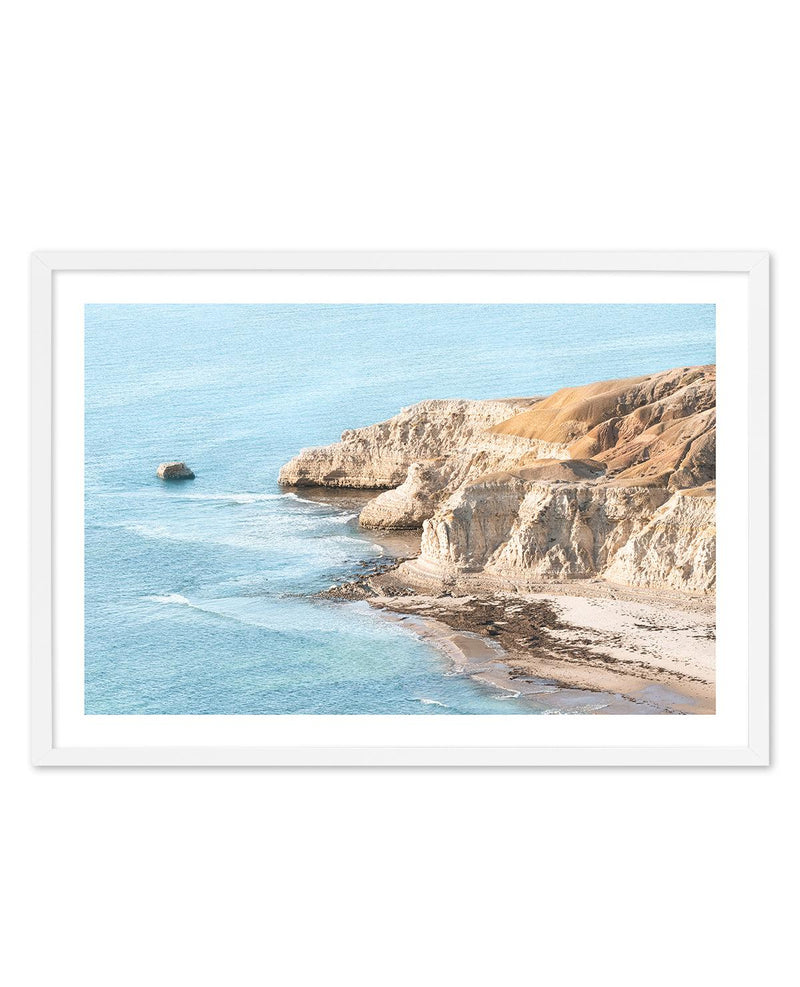This is a highly detailed landscape photograph, elegantly framed, depicting a coastal scene characterized by prominent cliffs and vibrant blue waters. The massive chalk-colored cliffs dominate the right-hand side of the image, suggesting their ancient geological origins judging by the visible stratification lines. These rugged formations, devoid of any greenery, extend right up to the water's edge, accompanied by a sense of solitude as the beach below remains completely vacant. The irregular shoreline shows signs of erosion, enhancing the raw, untouched beauty of the site. The blue ocean, shimmering with clarity and unique hues, teems with gentle waves lapping into the inlets between the cliffs. Additionally, there is a smaller, smoother outcropping of similar material perched in the water near the cliffs, adding another point of interest to this serene, uninhabited coastal environment.